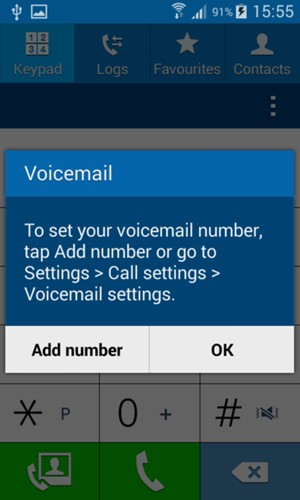The image displays a smartphone interface with a battery level of 90% and the time set to 15:55. The top of the screen features tabs: Keypad, Logs, Favorite Contacts, and Voicemail. The screen is currently focused on the Voicemail setup. Instructions are provided to set your voicemail number, offering options to "Add Number" or navigate to "Call Settings" and "Voicemail Settings" to add the number.

The lower portion of the interface includes two buttons: "Add Number" and "OK," written in black text on white background. The on-screen keypad is partially visible with keys for the star (*), zero (0), and pound (#) symbols. Additionally, some buttons for contact call options, call initiation, and a back function are present but not fully displayed. The primary colors used in the interface are blue, white, black, and green. The keypad has a gray overlay, while the popup dialog is presented in blue and white, providing clear step-by-step instructions for adding the voicemail number.